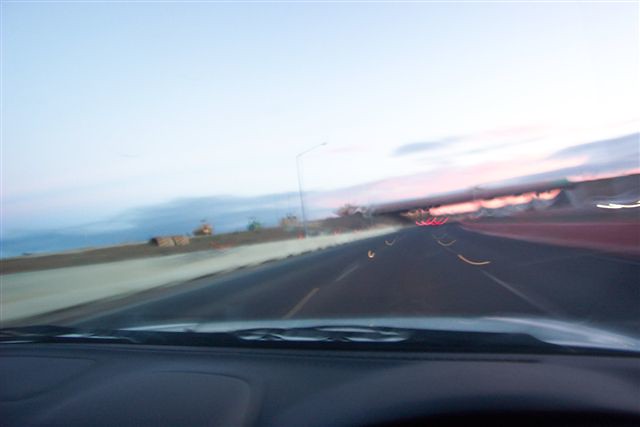The image captured is through the windshield of a moving car, giving a dash cam perspective with the dashboard and a windshield wiper partially visible at the bottom of the frame. The slightly blurred photograph shows an empty highway extending forward, with no other vehicles in close proximity. In the distance, a bridge is visible, appearing towards the far side, under which the road stretches. A series of red taillights faintly twinkle in the far distance near the horizon. It's during sunset, illuminating the sky with a beautiful gradient of light blue transitioning to a peach-pink glow near the horizon, especially towards the right side of the image, interspersed with some blue clouds. The scene is softly bathed in the warm hues of the setting sun. Additionally, a single street light stands on the side of the road, and a retaining wall can also be discerned in the background. The sky, though predominantly light blue, has some overcast regions mixed with visible clouds.